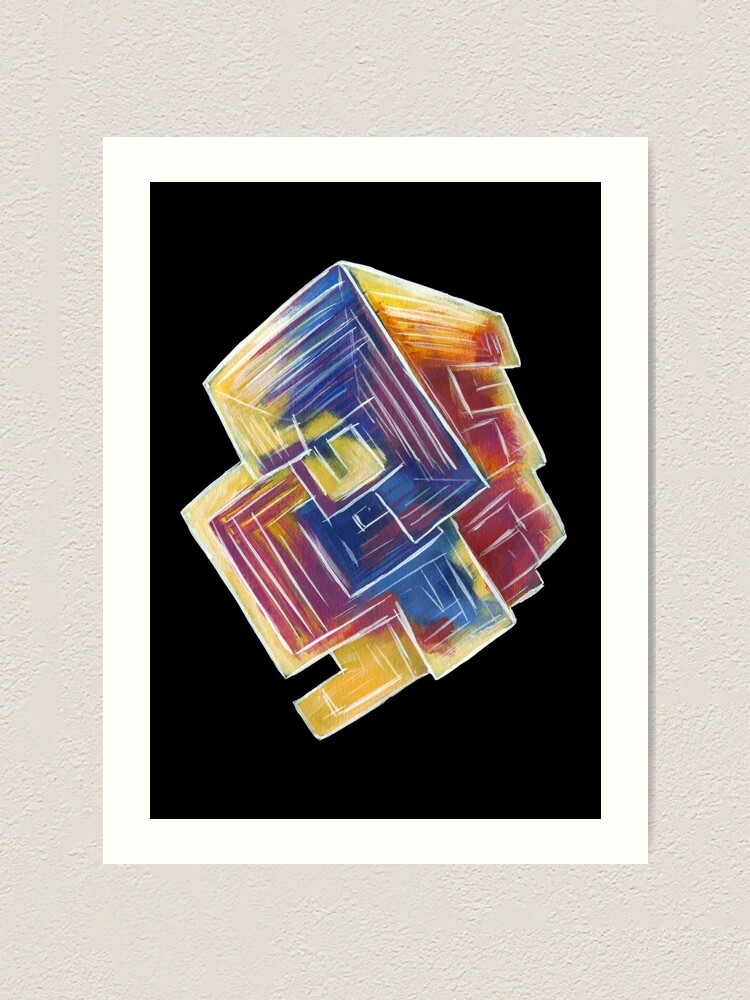The image shows a painting with an abstract structure at its center. It hangs on a wall that has a light gray or blue background, reminiscent of a stucco texture. The painting itself is enclosed in a smaller rectangular frame, approximately six inches high by four inches wide, with a half-inch thick white border. Inside this border, there's a black background on which the main subject is placed.

The central figure in the painting resembles a deconstructed Rubik's Cube with a highly irregular geometric shape, composed of interconnected and somewhat organic forms made predominantly of white lines. These forms create an intricate cuboid-like structure that has been shifted and rearranged in various sections, giving it a dynamic, almost three-dimensional appearance. The colors within this abstract arrangement include vibrant hues such as purples, reds, oranges, blues, and greens, strategically placed to enhance the visual complexity. Specific details like a backward C in yellow and a red C outline with yellow accents, along with red and orange striping, offer a vivid explosion of color, suggesting depth and movement within the piece.